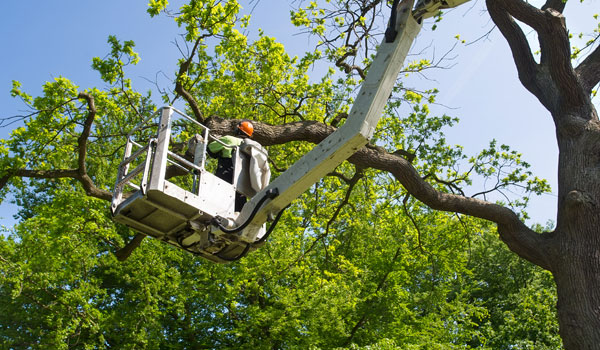In this image, the viewer's perspective is from the ground, pointing upwards. A muscular gentleman is elevated on a white scissor lift, also known as a cherry picker. The lift features a metal open-air platform designed for one or more individuals to stand in, operated either by controls on the platform or by someone on the ground. The man is wearing an orange hard hat and a green reflective jacket, indicating he may be working for the county or another public works entity. The backdrop includes a large tree abundant with green leaves, suggesting the season is either spring or summer. The clear blue sky enhances the bright, outdoor setting. The man's purpose on the lift could involve tree maintenance, perhaps trimming branches encroaching on power lines, although the specifics of his task are not evident from the image.